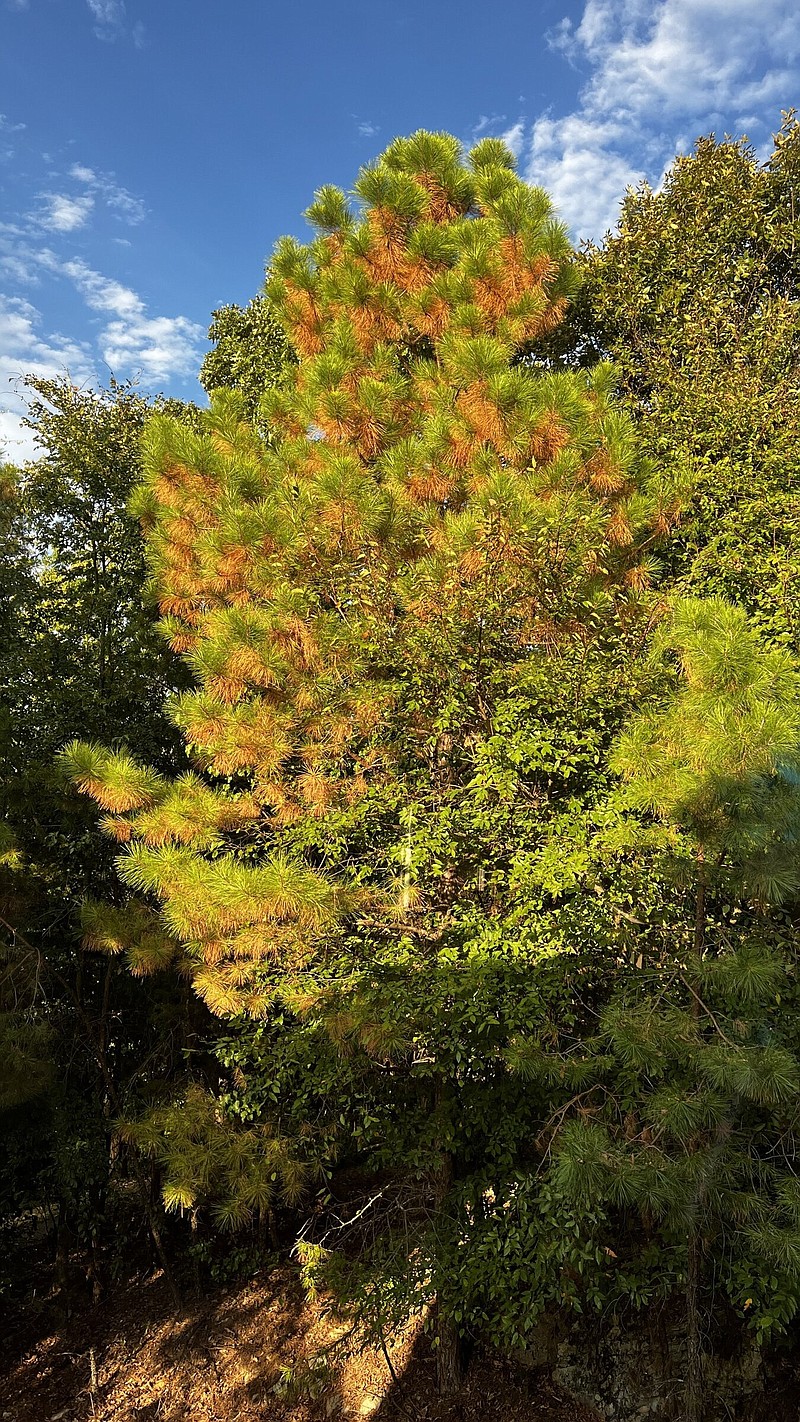The image captures a vibrant, sunny day in a forest with a large pine tree as the central focus. The towering pine tree, adorned with a mix of green and brown needles, stands prominently against a clear blue sky with wispy white clouds scattered across. This tree's significant height suggests its age and prominence in the forest. Surrounding it are various other trees with broad, green leaves, contrasting the pine. The bright sunlight illuminates both the pine tree and the forest floor, where dark shadows mingle with a carpet of brown soil, fallen pine needles, and leaves. The scene is devoid of any man-made objects or people, emphasizing the natural beauty and tranquility of this lush, green forest setting.